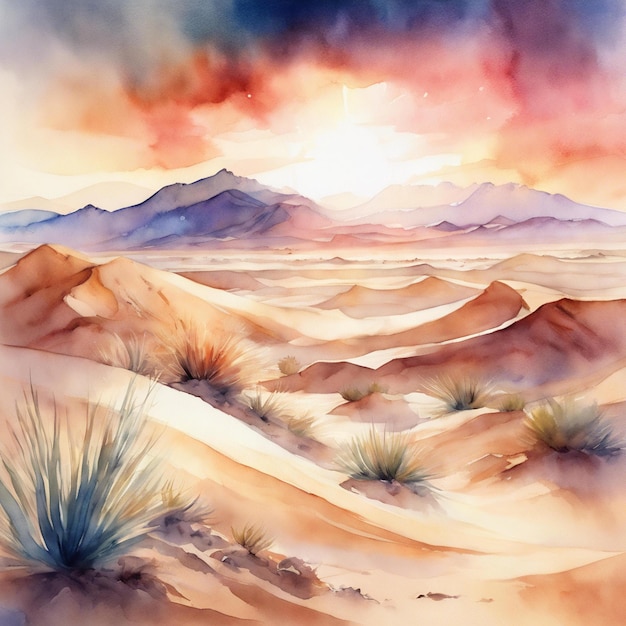This painting depicts an abstract desert landscape with an array of pastel and watercolor elements. In the background, tall, purplish mountains stretch across the horizon, tinged with shades of pink and brown. The sky above is a complex mix of colors—grey, blue, orange, pink, and reddish-purple—suggesting a dramatic sunrise or sunset. Bright white light in the center of the sky indicates the position of the sun. 

In the foreground, clusters of spiky grass dot the sandy terrain, which is primarily tan and light orange, interspersed with patches of brown. The sand appears windblown, forming dunes and small hills, adding texture to the barren landscape. Despite its minimalist and somewhat abstract representation, the painting vividly portrays an arid, desert environment devoid of people, animals, or man-made objects.